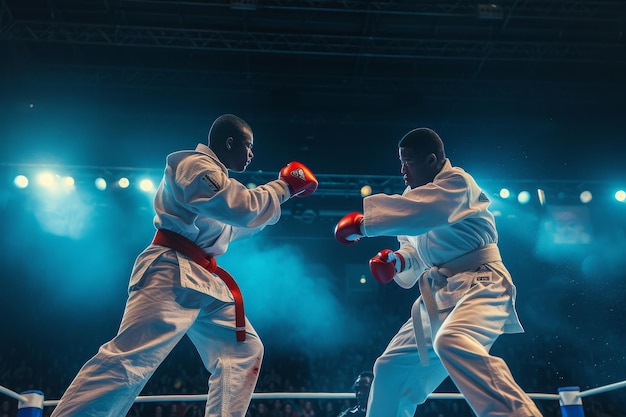This image captures a dynamic scene featuring two African-American men engaged in a boxing match within a brightly lit stadium. The focal point is the men who are standing in a boxing ring, both donning white gi-like robes. The man on the left is distinguished by a red belt and red and white boxing gloves, while the man on the right wears a white belt but matches his opponent with red and white gloves. Both are poised in a ready stance, facing each other in anticipation of the next move. Surrounding the ring, which is defined by white ropes and blue corner posts, a blurred crowd sits in the dimly lit background. Overhead, a series of bright lights illuminate the fighters, highlighting the intensity of the match in this dramatic, ground-level shot. An African-American referee can be faintly seen in the background, adding to the authenticity and tension of the moment.